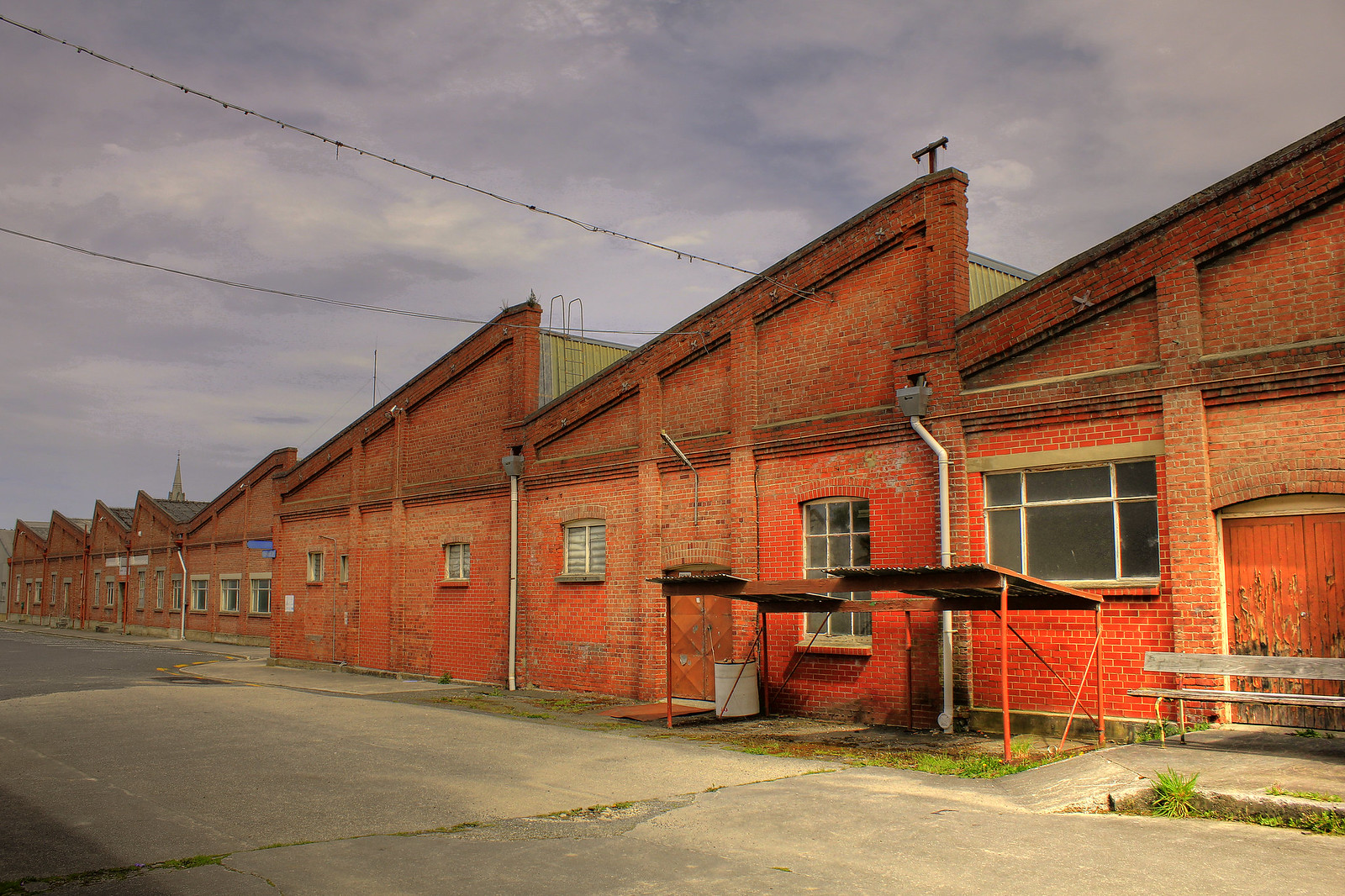The image depicts a row of brick buildings with slanted roofs, taller on the right side and shorter on the left, creating a repetitive, stepped pattern. The sky above is gray and cloudy, contributing to the overall faded or washed-out color tone of the image. Power lines are visible above the buildings, further enhancing the urban feel. Each building in the row is identical in shape but differs slightly in the number and size of windows. Some buildings feature three identical windows, while others have two or three of varying sizes. 

In front of the buildings, there is an empty parking lot, adding to the sense of openness in the foreground. Specific details of the scene include a small structure with orange poles and an aluminum-sheet roof on the farthest building to the right. Nearby, there is a white can, potentially a garbage can or barrel, and scaffolding beside a chair blocking the front door. Additionally, a bench is visible in front of one of the buildings, and yellow siding and a ladder are noticeable on one of the roofs. In the background, the steeple of a church can be seen, hinting at the surrounding neighborhood. 

The color palette includes shades of red, orange, green, blue, gray, and black, with no text present in the image. Overall, the scene is a cohesive blend of industrial and everyday urban elements under a somber, overcast sky.